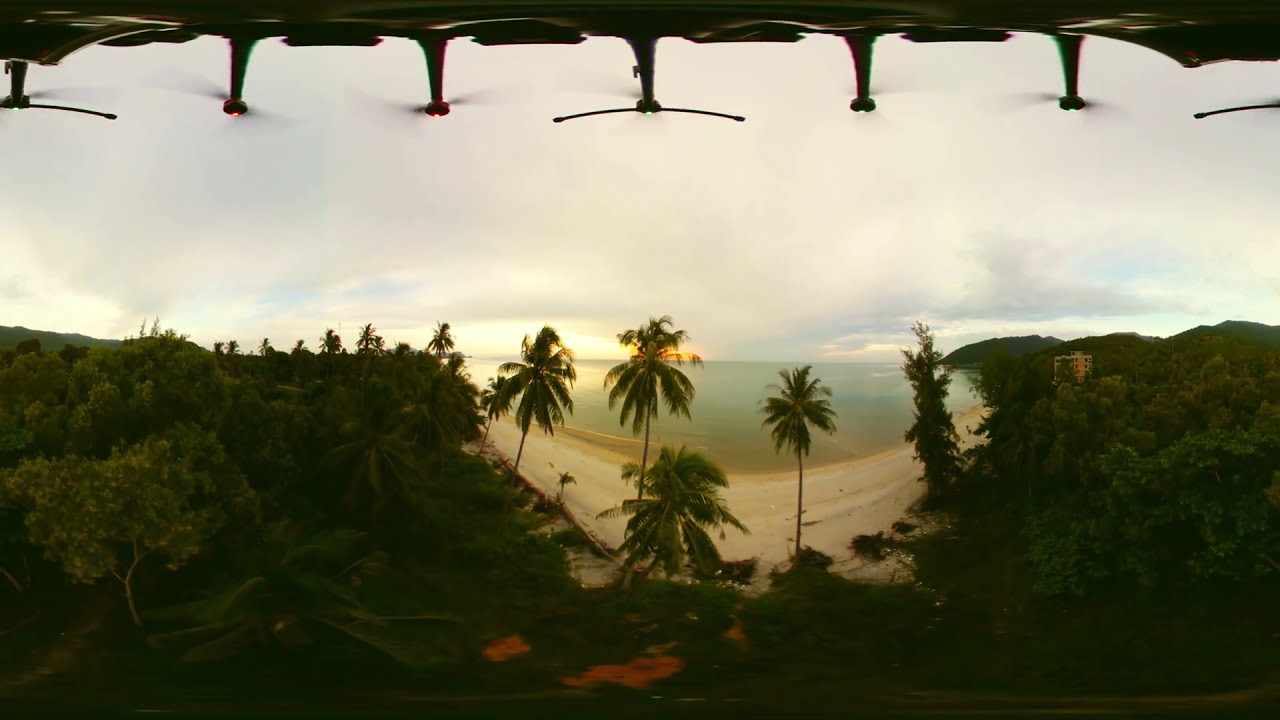The photograph is a rectangular image capturing a stunning tropical landscape, likely shot from a balcony or some elevated structure. At the top of the photo, partially visible ceiling fans or aerial propellers are spinning, adding a dynamic effect. The primary focus of the image is the lush, heavily forested, mountainous terrain covered in thick vegetation, resembling a tropical rainforest or jungle. 

At the center of this verdant scene stands a few tall, majestic palm trees, framed by dense foliage. The terrain creates a distinctive U-shaped hollow that leads to a serene, sandy beach. Beyond the beach lies a vast, crystalline turquoise ocean, its calm waters glistening under the muted light. The sky above is overcast with predominately gray and white fluffy clouds, though faint patches of blue sky peek through, hinting at clearer weather. The overall scene is tranquil and picturesque, resembling a secluded beach resort, free from any human presence.